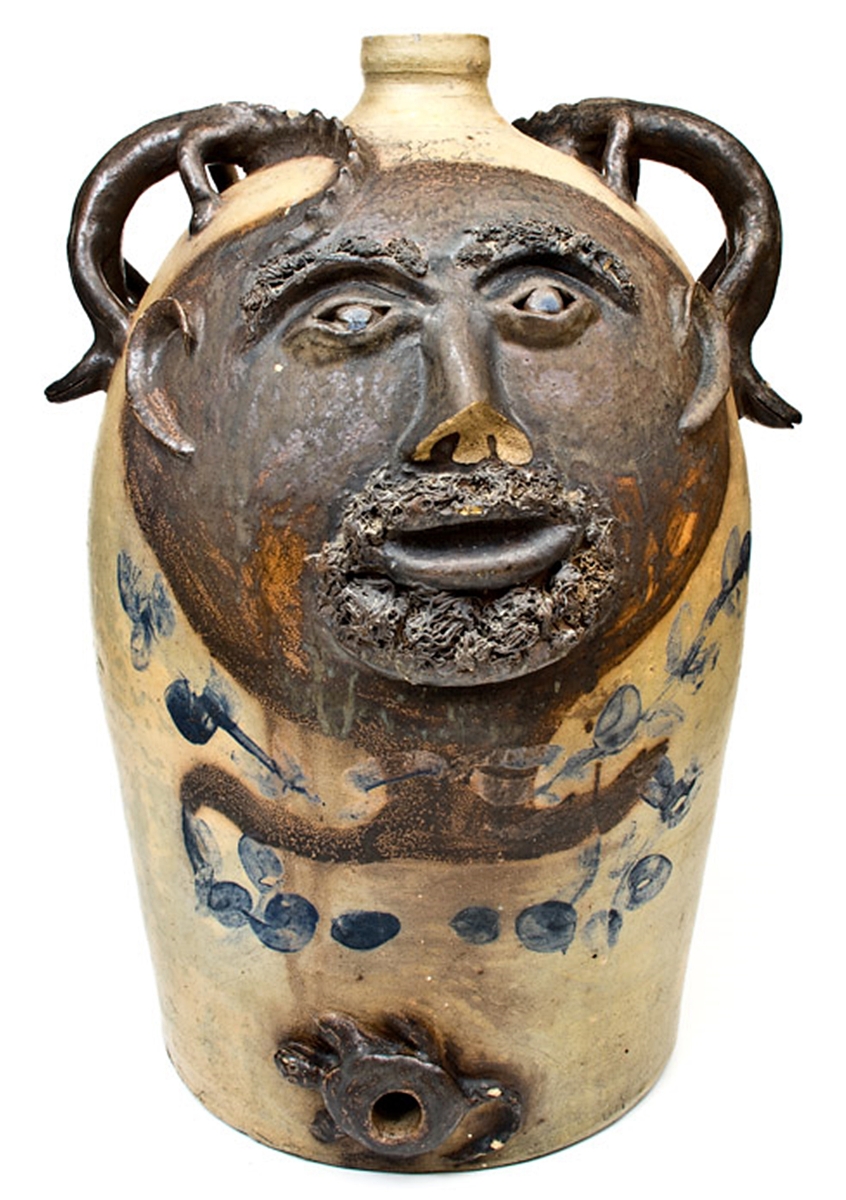The photograph depicts an ancient, wide-bodied ceramic jug with a small lip at the top, set against a plain white background. The jug, cream to beige in color, features an intricately carved dark brown face on the front. The face exhibits bushy eyebrows, deeply set eyes, and a textured mustache and goatee. The nose appears chipped, revealing the underlying lighter material. The face is adorned with crescent moon-shaped ears and a small, open mouth. 

The jug is decorated with random blue circles, vaguely resembling berries or floral patterns, scattered across its midsection. At the bottom of the jug, there is a small hole encircled by a dark gray, possibly turtle-like design. The jug's handles, dark brown and resembling either corns turned downward or ram's horns, are situated on either side at the top, merging seamlessly with the body. The overall aesthetic hints at a combination of rustic and mystical elements, with the jug's spout located centrally at the top. The entire artifact conveys a sense of aged artistry and enigmatic symbolism.